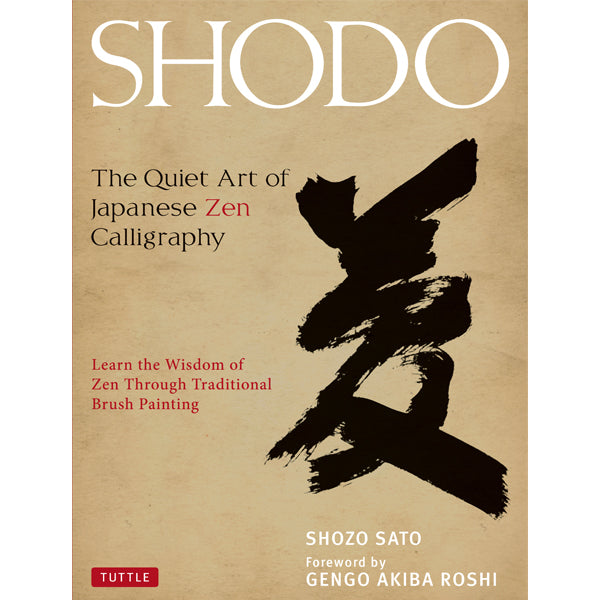The image displays the cover of a book titled "Shodo: The Quiet Art of Japanese Zen Calligraphy." The background features a beige, paper-like texture. At the top, "Shodo" is prominently written in large white letters. Below it, in black text, the subtitle reads "The Quiet Art of Japanese Zen Calligraphy," with the word "Zen" highlighted in red. Further down, in red text, it states "Learn the wisdom of Zen through traditional brush painting." The bottom left corner has a red box with white text that reads "Tuttle." On the right side of the cover, a black brushstroke kanji character is prominently displayed, providing a traditional touch. At the bottom right, in white text, it credits the author, Shozo Sato, along with a foreword by Gengo Akiba Roshi.